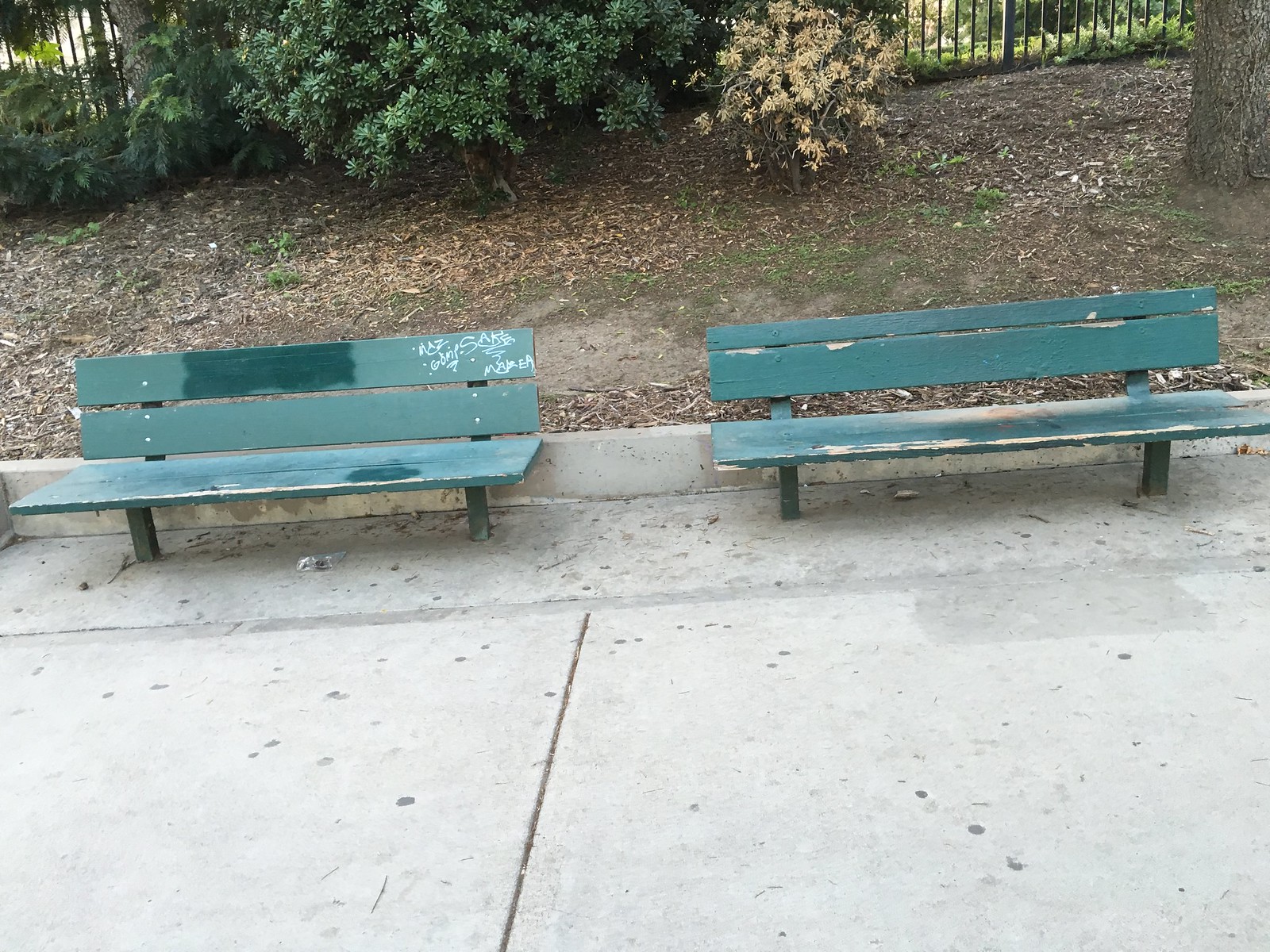The image depicts an outdoor scene featuring two green wooden park benches set on a concrete sidewalk and curb that take up the bottom half of the image. The benches are made from board planks with two legs on each and are notably worn, showing exposed wood in several places due to chipping paint. The bench on the left has visible white graffiti on its top right seating area and multiple patches of darker green paint covering up previous graffiti, while the bench on the right appears even more worn with significant areas of exposed wood. The concrete path in front of the benches is littered with debris and hardened black gum stains. Behind the benches is a messy hillside covered with twigs, dead leaves, and plant debris, leading up to an iron fence at the top of the hill. In front of the fence, on the right side of the image, there are a few large shrubs and a tree, adding to the disordered backdrop.